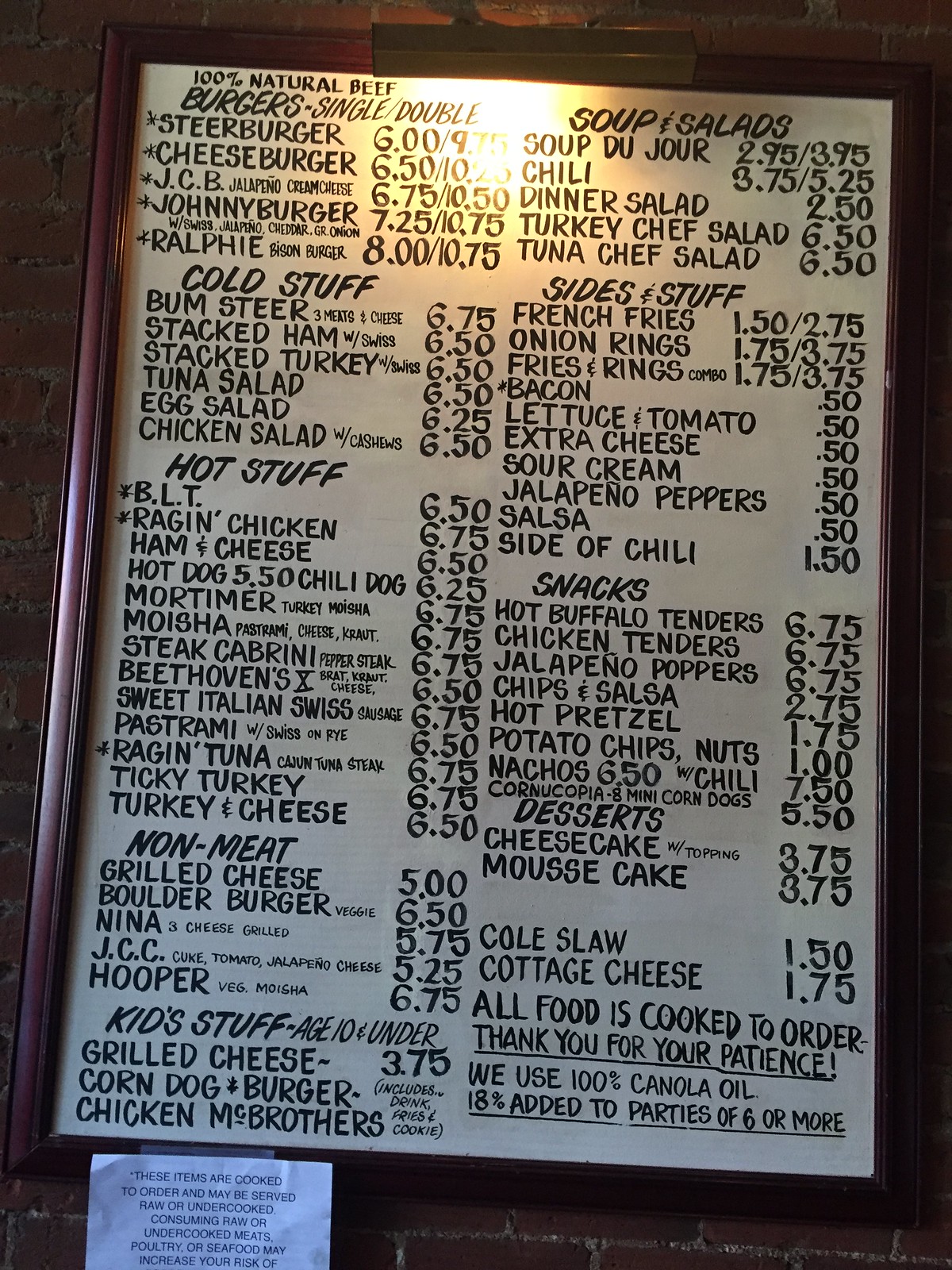A detailed menu is prominently displayed on a whiteboard framed by dark wood with a thin border. The frame, mounted against a red brick wall, is illuminated from above to enhance visibility. The extensive menu is divided into sections, each heading written in capitalized italics, showcasing a wide array of items listed underneath in capitalized non-italics. Each menu item is accompanied by its price, with some featuring additional pricing for single or double portions. At the very top, a header clarifies the pricing structure. Below the whiteboard, a white piece of paper is taped on, cautioning patrons that "These items are cooked to order. It may be served raw or undercooked. Consuming raw or undercooked meats, [portion of your seafood may increase your risk of]" before the message cuts off. The menu categories include Burgers, Soups and Salads, Sides, Hot Stuff, Cold Stuff, Snacks, Non-Meat, and a Kids Menu, offering a diverse selection to satisfy various tastes.